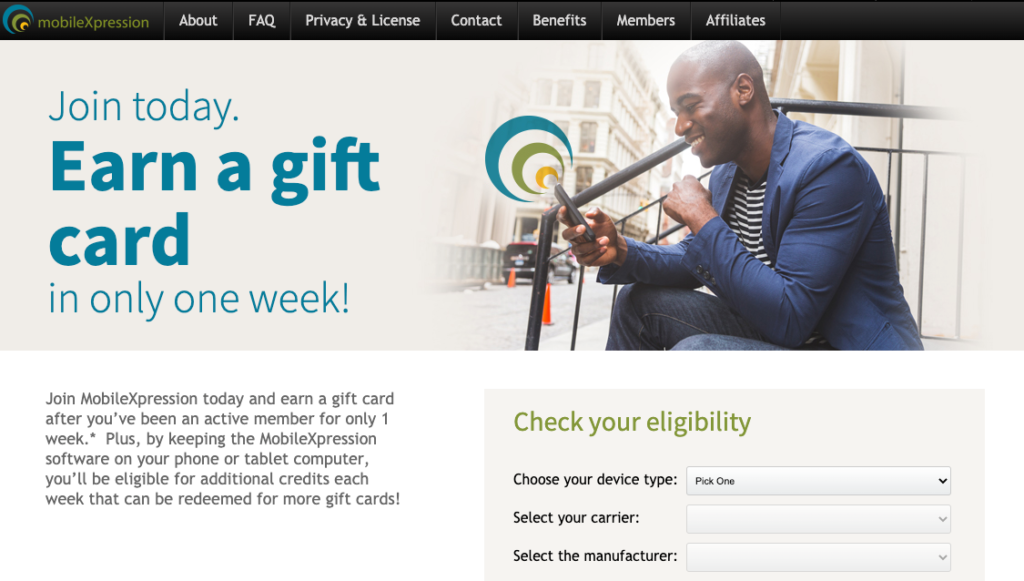The website for Mobile Expression features a vibrant logo with multi-colored symbols in gold, gray, and blue, radiating outward like waves. The top navigation bar is black, offering links to various sections such as About, FAQs, Privacy and License, Contact, Benefits, Members, and Affiliates. The background of the homepage is an understated, off-white shade, providing a clean canvas for the text on the left side.

Highlighted in a teal blue regular font are the words "Join today," followed by a bold statement "Earn a gift card" in larger text, and an additional line in the original font stating "in only one week." 

To the right of this text, there is an image of a well-dressed man sitting on his front stoops, set against a city backdrop. He is wearing a blue blazer over a blue and white horizontally striped shirt and jeans. The man is happily engrossed in his phone, with symbols emanating from the device, suggesting activity or connectivity. A handrail is visible behind him, adding to the urban setting.

Below this, a white bar spans the width of the section. On the left side, a paragraph encourages users to "Join Mobile Expression" and "earn a gift card after being an active member for only one week," indicating an opportunity for quick rewards. An asterisk hints at further details available elsewhere on the site.

To the right, a green box allows users to check their eligibility. The box, set against an ivory-colored background, prompts users to choose their device type, carrier, and manufacturer. Upon confirmation of eligibility, users can begin earning money through the platform.